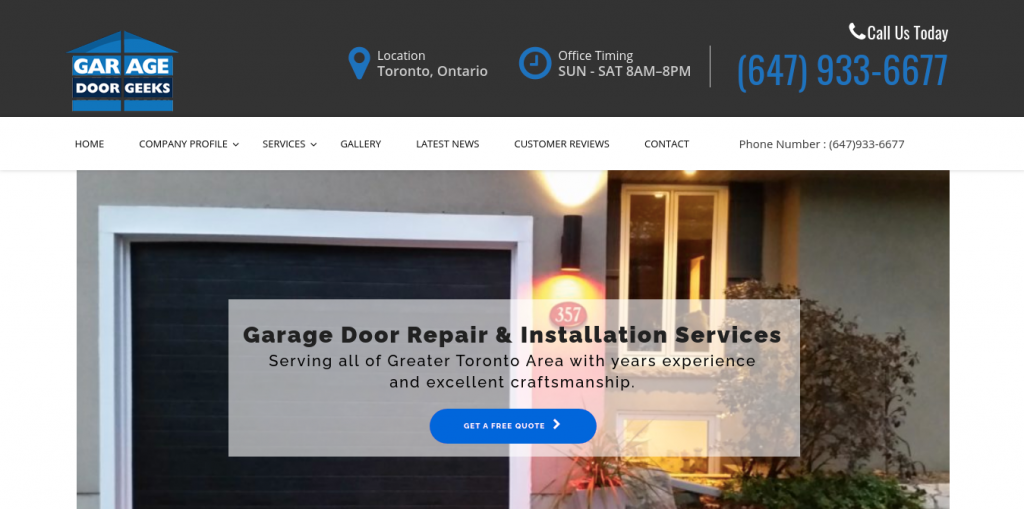The screenshot showcases the homepage of a website called "Garage Door Geeks," which appears to be a business specializing in garage door services. The website features a logo consisting of white text over a blue background in the shape of a simple house or possibly a freestanding garage. The header of the page is gray, marked by the business name and a location pin specifying "Toronto, Ontario." Adjacent to the location information, there is a clock icon indicating the office hours, which are Sunday through Saturday from 8 a.m. to 8 p.m. On the right side of the header, there is an option to call the business, "Call Us Today," featuring the phone number 647-933-6677 in white text. 

Beneath the header, a navigation menu includes sections for "Home," "Company Profile," "Services," "Gallery," "Latest News," "Customer Reviews," and "Contact," with the phone number displayed again.

An image occupies the central portion of the page, depicting a simple gray house with the house number "357" above a black garage door framed in white. A black tube sconce is mounted above the house number, emitting light both upward and downward. 

Overlaying the image is a translucent white panel with black text that reads: "Garage door repair and installation services. Serving all of Greater Toronto area with years of experience and excellent craftsmanship." Below this text, a blue, capsule-shaped call-to-action button invites users to "Get a free quote," accompanied by an arrow on the right side.